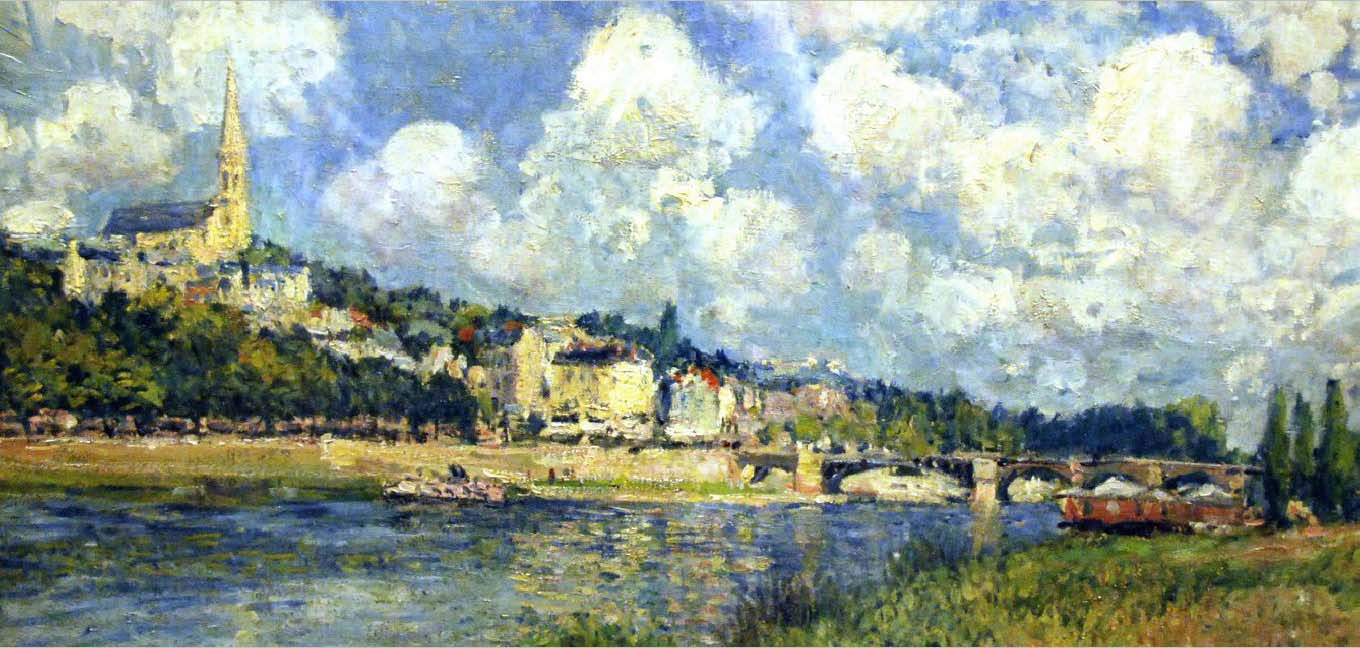This is a detailed, brightly colored oil painting that captures a picturesque landscape of a serene, coastal village. The painting is oriented in landscape format and features a vibrant, blue river running through the middle, reflecting the vivid colors of the surrounding scenery—golds, greens, and yellows dancing on the water's surface. On the right side of the image, a charming arched bridge connects the foreground to the village across the river. 

The lower right corner of the painting reveals a grassy waterfront area, dotted with trees. The village, nestled on the side of a gently sloping hill, is crowned by an imposing church with a tall yellow spire and a gray roof. The village buildings, adorned with bright, colorful roofs in shades of red, cream, blue, and gray, cascade down the hill, surrounded by lush greenery of trees and shrubs.

In the background, a mostly blue sky is accented by clusters of thick, white, puffy clouds, adding to the painting's overall serene and idyllic atmosphere. The bridge in the background on the right side of the painting leads to this enchanting village, further enhancing the sense of connectivity and charm. The combination of these elements—the tranquil river, vibrant architecture, and lush natural surroundings—makes for a very pleasing and detailed depiction of a quaint, lakeside or canal-side village.